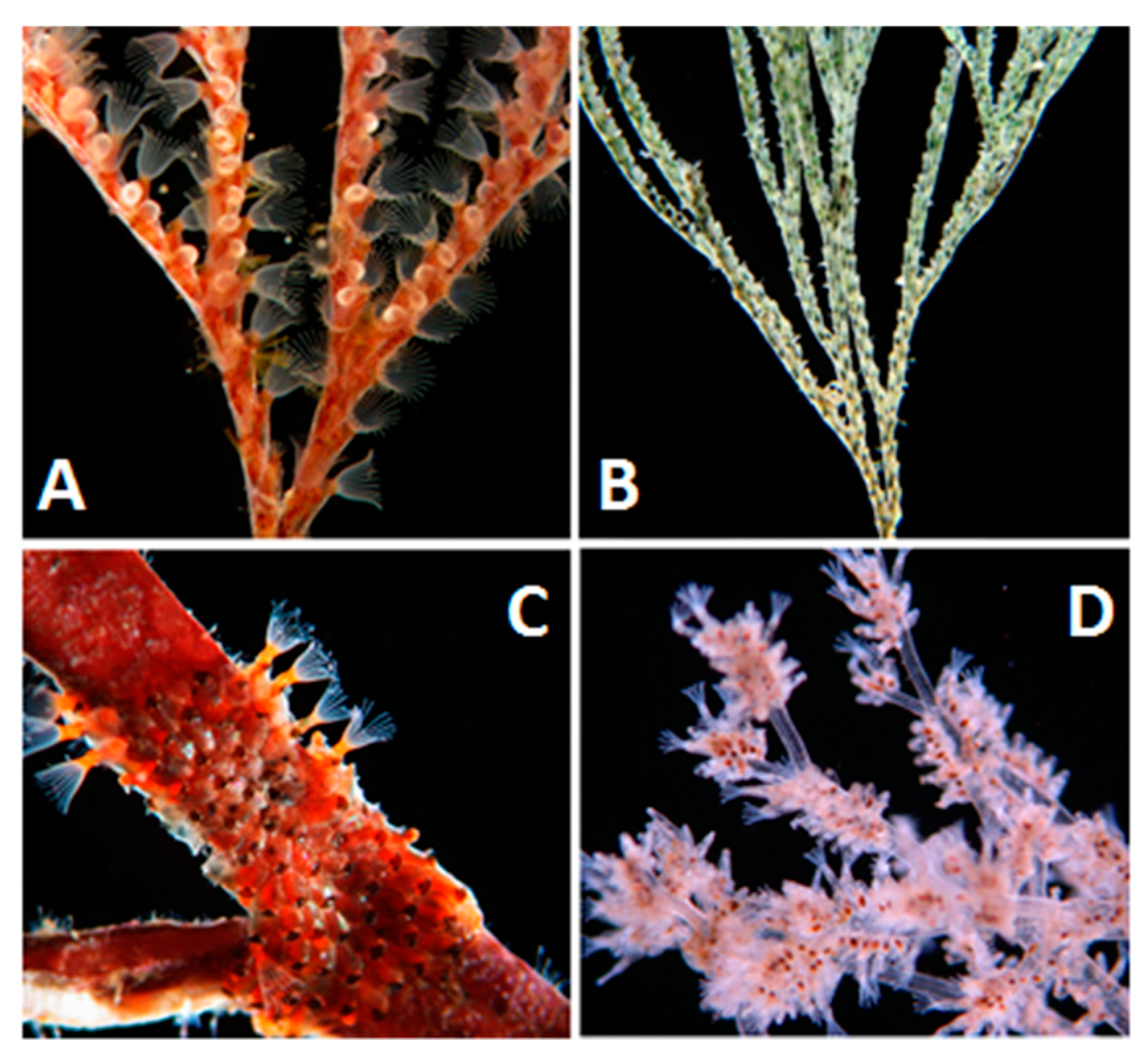This detailed scientific photograph is divided into four quadrants, each showcasing a different type of bryozoan, all set against a black background with a white cross separating the sections. The top left quadrant features bryozoan "A," which is a long, bright red specimen with white and clear cup-like structures adorning its sides. It resembles an orange plant with tiny, wing-like extensions. The top right quadrant displays bryozoan "B," characterized by its elongated, stem-like appearance and a mixture of white, green, and yellow colors, giving it a spiny and rough texture. The bottom left quadrant contains a close-up of bryozoan "C," a thicker, reddish organism with fewer small white cups and some feathery, hair-like sections protruding. Lastly, the bottom right quadrant shows bryozoan "D," distinct in its clear, branching structure with numerous frilly, pinkish-white cups, producing an appearance somewhat akin to a plant with white and red flowers. Each quadrant vividly illustrates the diverse morphology of these fascinating undersea or microscopic creatures, offering a detailed glimpse into their varied forms.